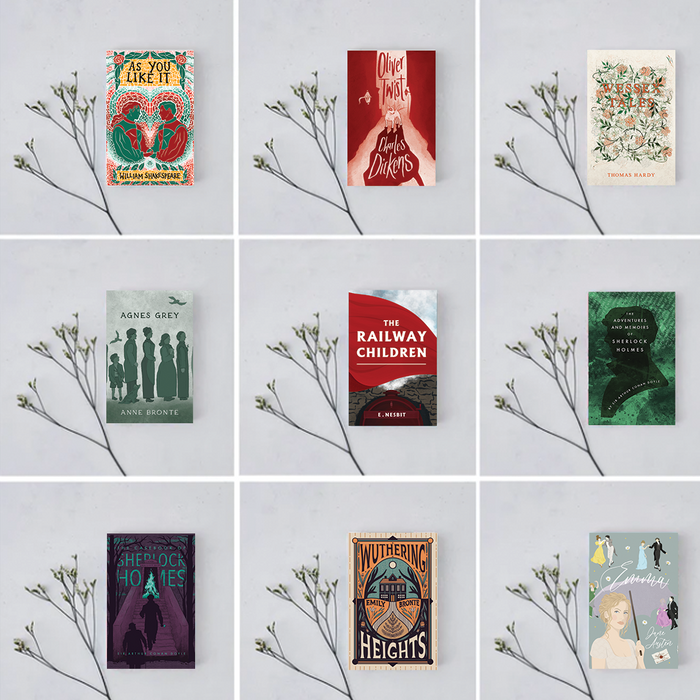The image consists of a square collage with nine individual squares arranged in a 3x3 grid on a light gray background. Each square displays a book situated to the right of a small, sparse tree branch or twig with tiny leaves or buds. The top row features "As You Like It" by William Shakespeare, "Oliver Twist" by Charles Dickens, and "Wessex Tales" by Thomas Hardy. The middle row showcases "Agnes Grey" by Anne Brontë, "The Railway Children," and "The Adventures and Memoirs of Sherlock Holmes" by Arthur Conan Doyle. The bottom row includes another Sherlock Holmes book, "Wuthering Heights" by Emily Brontë, and "Emma" by Jane Austen.